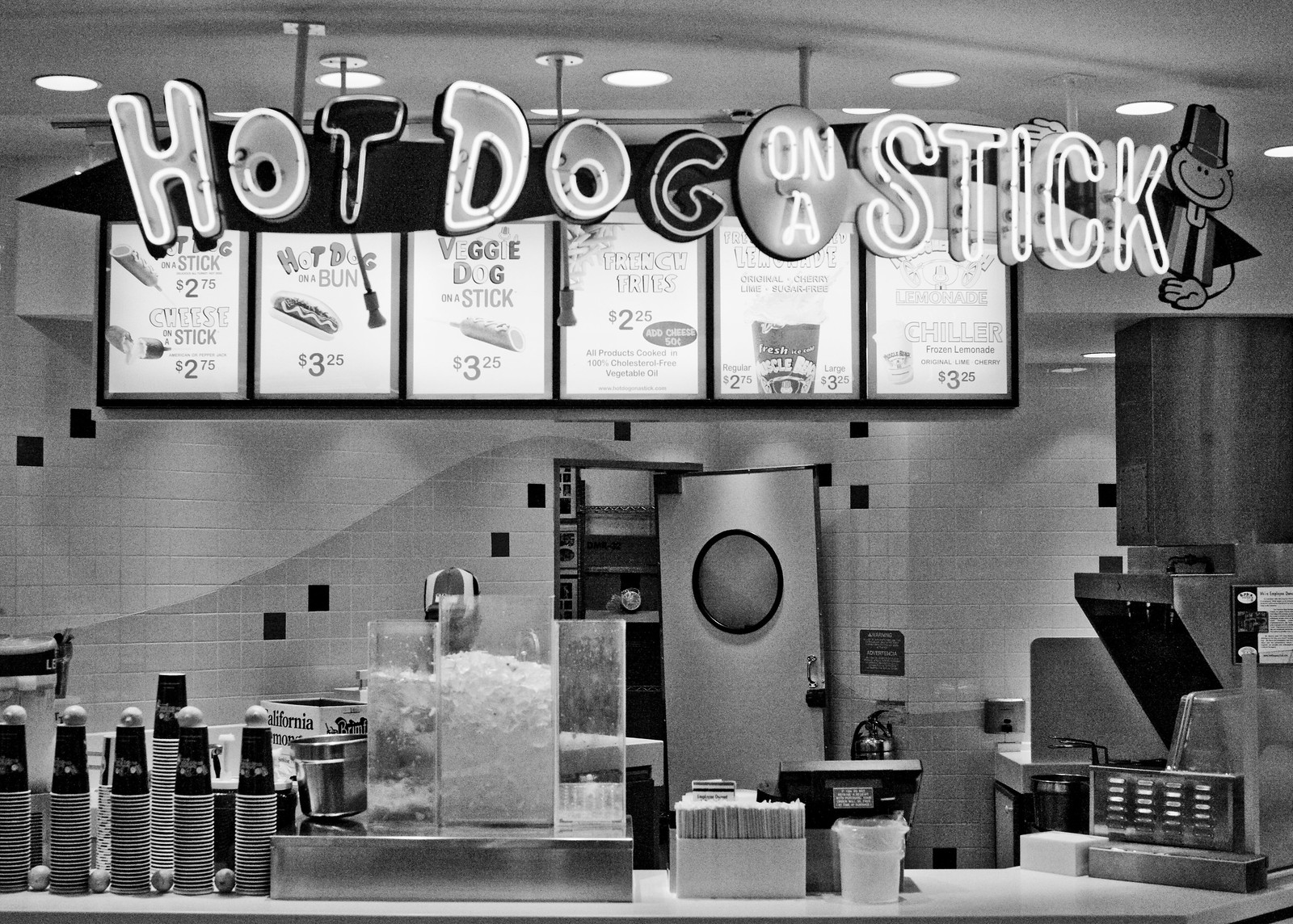This black and white photo captures an older-style, counter-service restaurant, prominently featuring a "Hot Dog on a Stick" neon sign above the service area. The black and white image reveals a classic eatery setup with an array of items typically found in such establishments. The counter is visible at the bottom, with stacked cups on the left side and ice and drink dispensers nearby. There is also a small bucket for tips next to the cash register. The right side of the photo includes various cooking equipment, including a fryer.

The menu is displayed above the counter in six distinct boxes, listing options that include a hot dog on a stick and a cheese stick both priced at $2.75, a hot dog on a bun for $3.25, a veggie dog on a stick for $3.25, French fries for $2.25, and lemonade chiller for $3.25. Illustrations of a character with a smiley face and a hat in a striped shirt adorn the signage, adding a nostalgic touch. In the background, an open door with a circular window leads to what appears to be the storage or cooking area. The wall behind the counter is tiled in white with occasional black tiles creating a diagonal pattern. The absence of people in the photo gives it a still, timeless quality, presenting a moment frozen in this quaint, monochromatic restaurant scene.